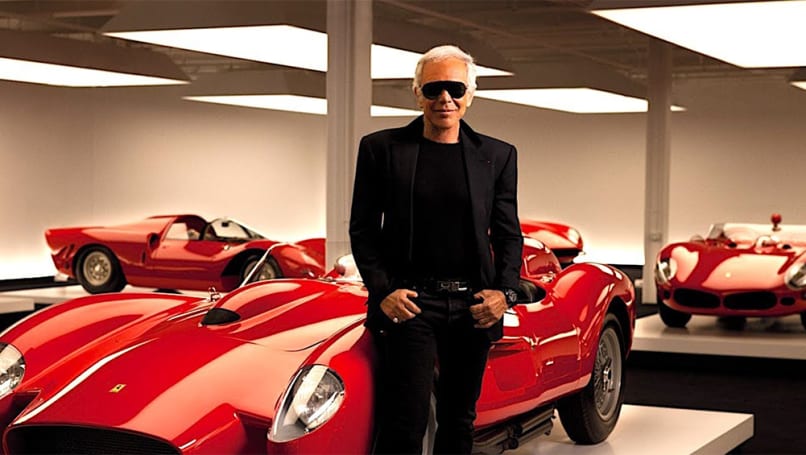In this photograph, a distinguished man with gray hair, black sunglasses, and a stylish all-black ensemble, consisting of a black blazer, shirt, and pants, is smiling directly into the camera. The backdrop reveals an opulent indoor setting resembling a high-end showroom or possibly a lavish car lot. Prominently displayed on various white platforms made from a grayish-tan material are four cherry-red sports cars, likely Ferraris or Bugattis, each gleaming under the showroom lights. The ceiling, painted black, features large light panels illuminating the scene. Two structural posts or pillars support the ceiling in the center of the room, adding to the sophisticated atmosphere. The luxurious environment suggests the man could be someone of notable wealth, confidently posing next to these elite convertibles.